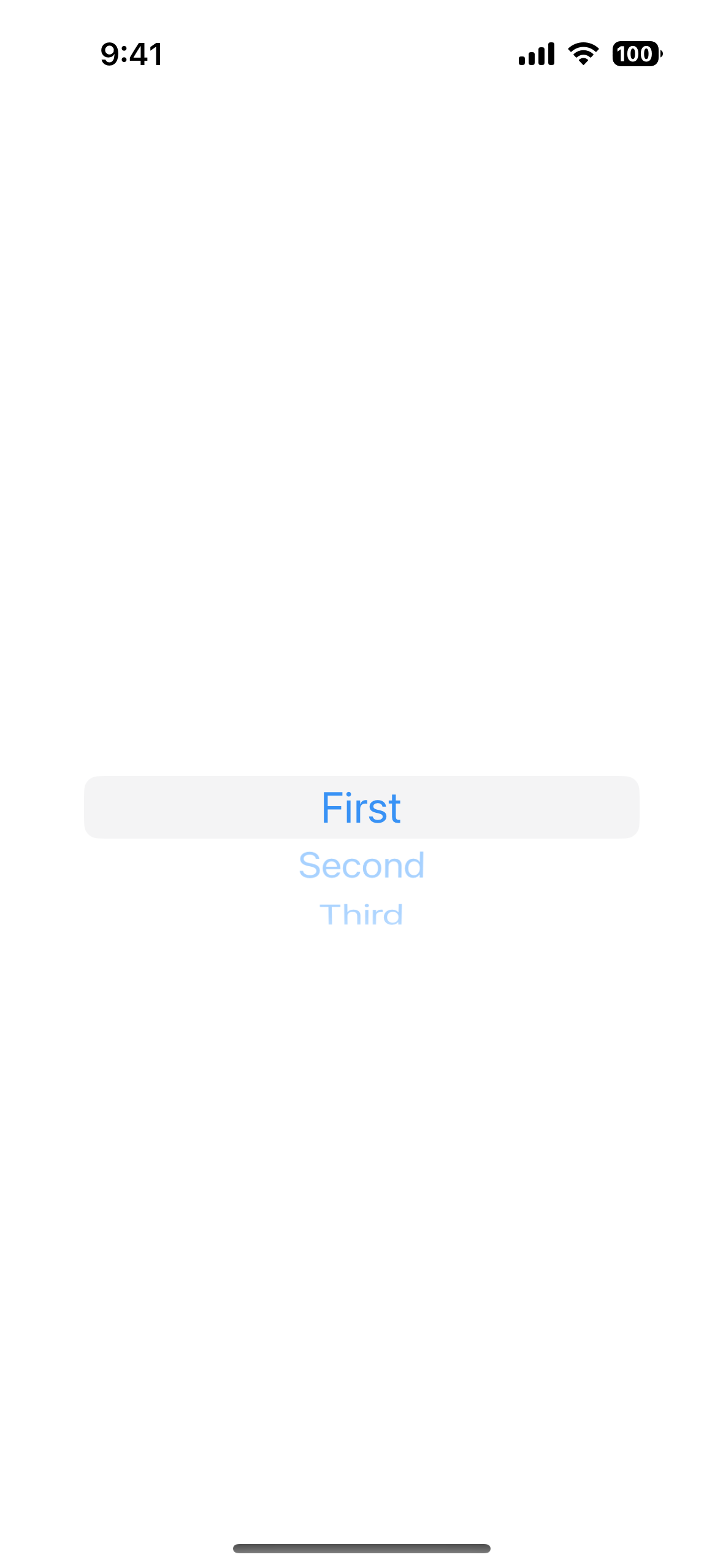The image is a vertical, borderless screenshot, likely captured from a smartphone, given its proportions. The background is entirely white, with essential status indicators at the top. In the top-left corner, the time is displayed as "9:41" in black text. To the right, there are four black signal bars of increasing height, followed by a Wi-Fi icon and a battery icon showing "100" in white text against a black background.

Dominating the center of the image is a very light gray horizontal rectangle. Inside this rectangle, "first" is centered and displayed in large blue text. Below "first," the word "second" appears in a lighter, faded blue. Directly underneath "second," the word "third" is present, though the very bottoms of the letters in "third" are slightly cut off, suggesting cropping. 

The bottom section of the image features a somewhat thick, dark gray horizontal line that spans the width of the image, positioned centrally at the bottom.